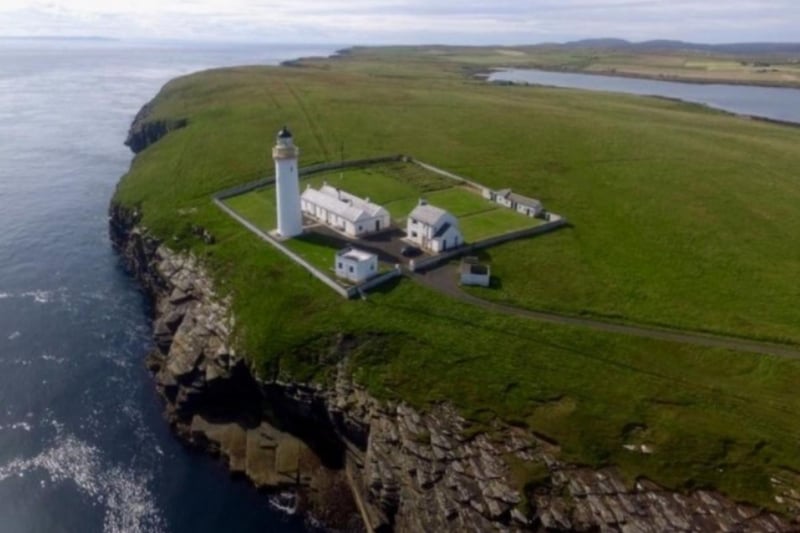This detailed aerial photograph captures a coastal scene dominated by a central lighthouse compound perched on a sheer gray stone cliff, enveloped by a lush expanse of short green grass. The image is rectangular, with the top and bottom edges twice the length of the left and right sides. At the heart of the image is a large, square-shaped compound, enclosed by a low white wall. Inside the compound, several white buildings are arranged around the striking lighthouse, which features a tall white tower topped with a conical black roof.

Among the buildings, a notable two-story structure near the front gate stands alongside a square-shaped single-story building. A long, barrack-style building with a sloped roof stretches out within the compound, reminiscent of a motel or a place to stay. Outside the wall, a wide asphalt road winds its way from the compound towards the right side of the photograph, eventually disappearing into the distance.

The cliff beneath the grass sharply descends to a stretch of dark blue water that hugs the left edge of the image. In the distance, the waterway extends into the background, bordered by faint mountains, while the sky above remains overcast with a thick layer of gray clouds, though there is no indication of rain. Overall, the scene depicts a serene yet rugged coastal landscape, punctuated by the historical and functional presence of the lighthouse and its surrounding structures.